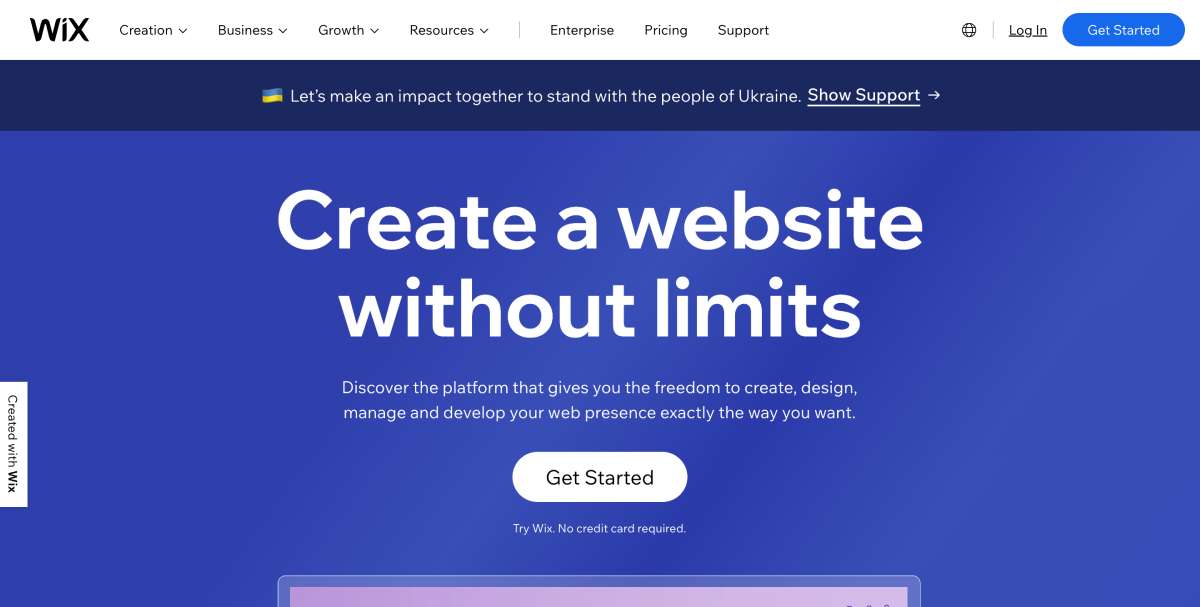The top portion of the image features a white background with the "Wix" logo in navy blue, followed by several navigational tabs: "Creation," "Business," "Growth," "Resources," "Enterprise," "Pricing," and "Support." A small black globe icon with an underline labeled "Sign In" appears, along with a blue button labeled "Get Started" in white font.

Beneath this, there's a navy blue rectangular banner displaying the Ukrainian flag on the left. The flag has a blue upper half and a yellow lower half. Accompanying text in white reads: "Let's make an impact together to stand with the people of Ukraine." Another clickable text in white and underlined says "Show Support" on the right.

Below this, there is another navy blue banner with white text saying "Create a website without limits." Additional white text directly below states: "Discover the platform that gives you the freedom to create, design, manage, and develop your web presence exactly the way you want." Within an oval outlined in white, "Get Started" is written in black font. Following this, in smaller white text, it reads: "Try Wix. No credit card required."

In the middle bottom section of the image, a partially visible area with hints of purple and bordered by another shade of purple is seen on the left edge. The bottom of the white rectangular section displays the text in black: "Create it with Wix."